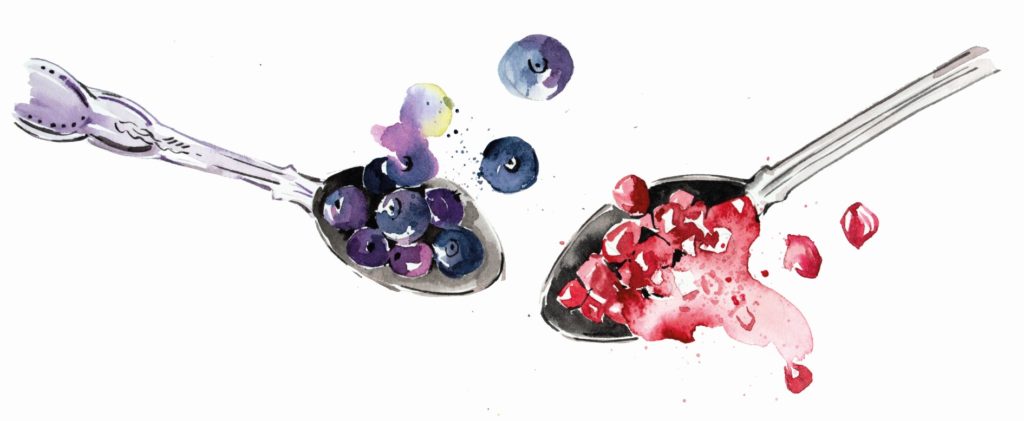The image is a digital-generated artwork featuring two intricately designed silver spoons set against a pristine white background scattered with colorful dots that represent the fruits. The spoon on the left, showcasing an ornate handle with purple hues, is cradling dark blue-purple blueberries that exhibit subtle yellow and white highlights. Some of these blueberries appear to be almost popping off the spoon, adding a dynamic touch to the artwork. The spoon on the right, which also has a detailed handle albeit with a more rounded design, contains vibrant red berries, possibly pomegranate seeds, with a hint of juice that seems to be bursting forth. The overall composition of the photo is vibrant and lively, highlighting the contrast and richness of the fruit colors against the minimalist backdrop.